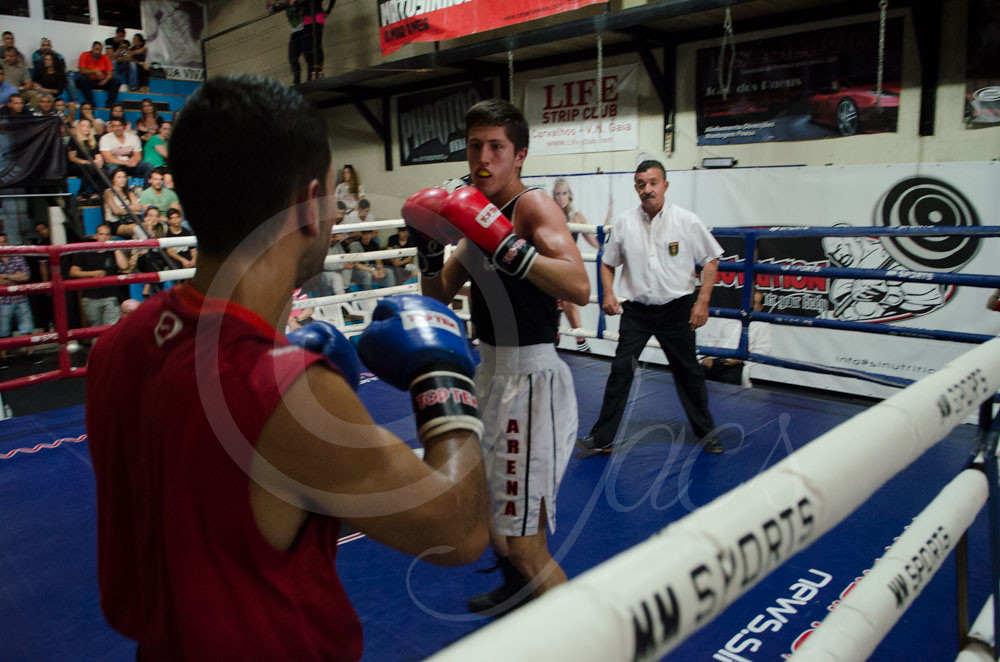The image captures an intense moment during a boxing match with two fighters prominently featured in the ring. The fighter facing the camera wears red boxing gloves adorned with a black design around the wrist and forearm. His mouth is slightly open, revealing a yellow mouth guard, and he is geared up in a black tank top and white gym shorts with the word "Arena" inscribed in red text. Across from him, with his back to the camera, is his opponent, sporting blue boxing gloves and a red sleeveless top. Both fighters, with short black hair, are in a ready stance with their fists up, indicative of the high-energy bout.

In the background, the referee, an older man with a mustache and black hair, dressed in a white button-up shirt and black pants, attentively watches the fighters. The ring's floor is blue, and its edges are lined with red, white, and blue ropes. The white cushioned corners bear the logo "MM Sports." Surrounding the ring, a captivated audience observes from the blue-toned stands, adding to the vibrant atmosphere of this dynamic scene.